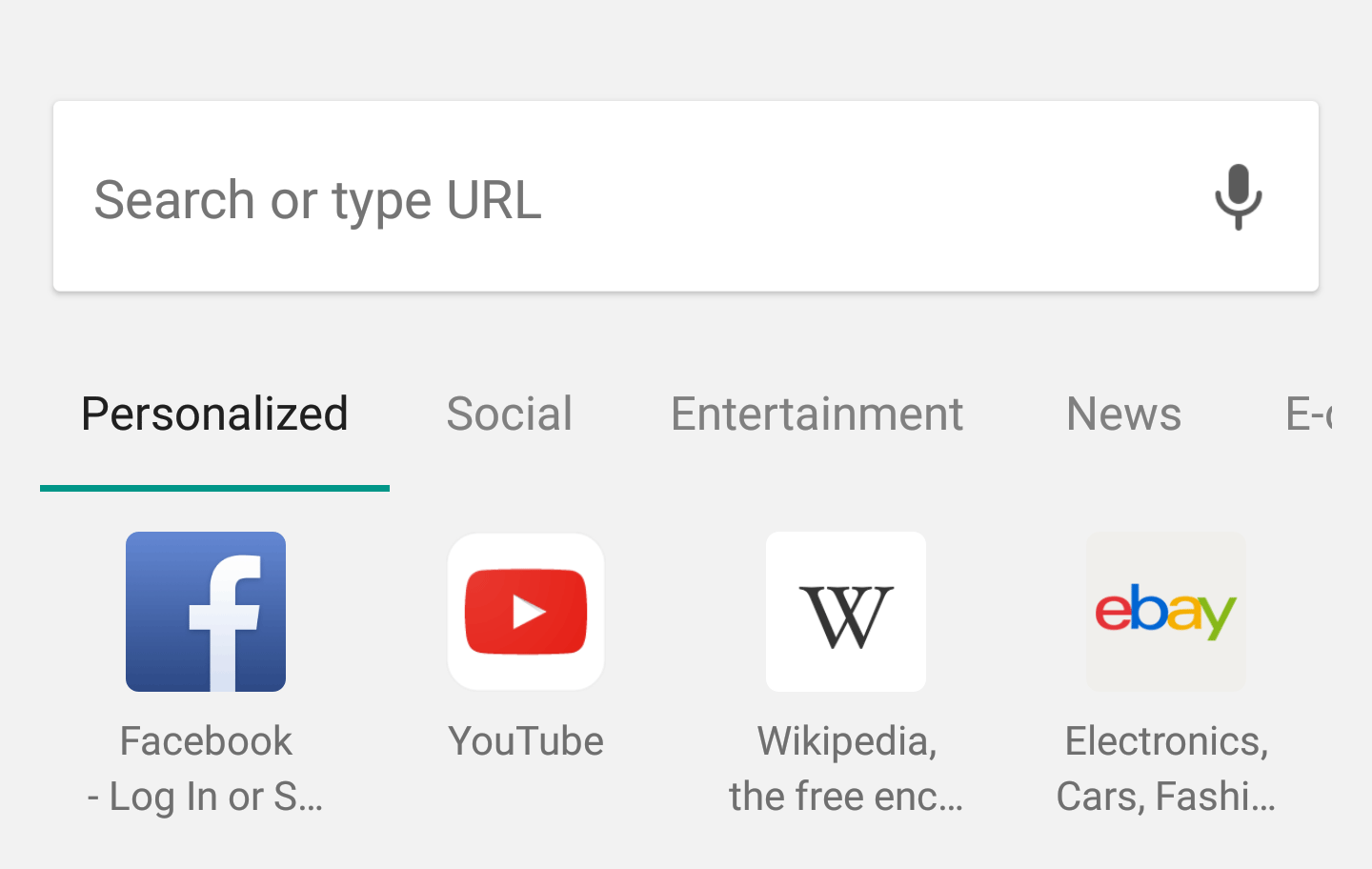The image appears to be a magnified screenshot of a browser window, showcasing various elements in detail. At the top of the screenshot, there's a light gray rectangle area containing a search bar set within a larger white box. The search bar has the placeholder text, "Search or type URL," and features a small microphone icon on its right side, likely indicating voice search functionality.

Below the search bar, there is a navigation menu with several tabs. The "Personalized" tab is highlighted in bold and underscored with a green line. Next to it, other tabs include categories such as "Social," "Entertainment," "News," and an incomplete one labeled "E..." which is cut off.

Further down, there are four square icons representing various websites. The first icon is blue with a white lowercase "f," indicative of Facebook, and is labeled "Facebook log in or s..." with the rest of the text cut off. The second icon is a white square with a red rectangle and white play button, labeled "YouTube." The third icon is a white square featuring a stylized "W," labeled "Wikipedia common the free ENC...," also cut off mid-sentence. Lastly, there is a light gray square labeled "eBay," with text indicating product categories like "electronics, cars, FSH IO..."

The entire screenshot appears to be zoomed in considerably, resulting in very large and partially cut-off text and icons, suggesting the intent to show details closely.